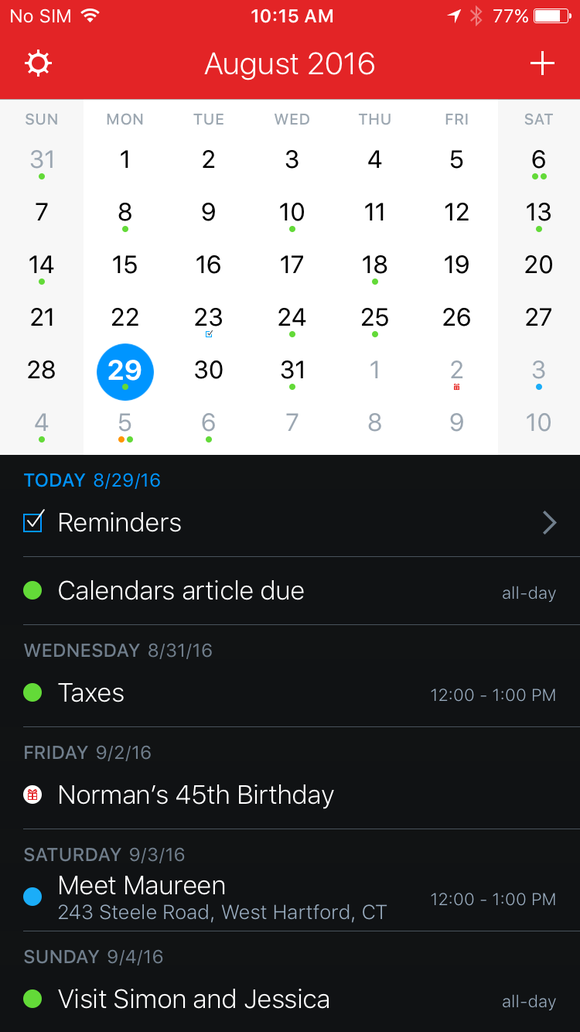In this image, we are looking at a screenshot of a smartphone interface. The upper left corner features a red header with white text indicating "No SIM." To the right, there is a Wi-Fi icon, followed by the time displayed as 10:15 AM in the center. Continuing to the upper right corner, there's a battery icon showing 77% charge, adjacent to an unlit Bluetooth icon.

The central part of the screen reads "August 2016" with a sun-like icon on the left and a plus sign icon on the right. Directly below this is a white calendar for August, with Monday the 29th distinctly highlighted in a blue circle.

Below the calendar, against a black background, the date is reiterated in blue text reading "Today, 8-29-16." Underneath, we see a section labeled "Reminders" in white text, accompanied by a white checkmark on the left and a right-pointing arrow on the right.

Further down, next to a green circle, is a list item labeled "Calendars," followed by the word "Article" and "Due." The next section indicates "Wednesday, 8-31-16" with a green bullet point. Adjacent to this, the text "Taxes, 12-1 PM" is displayed in white.